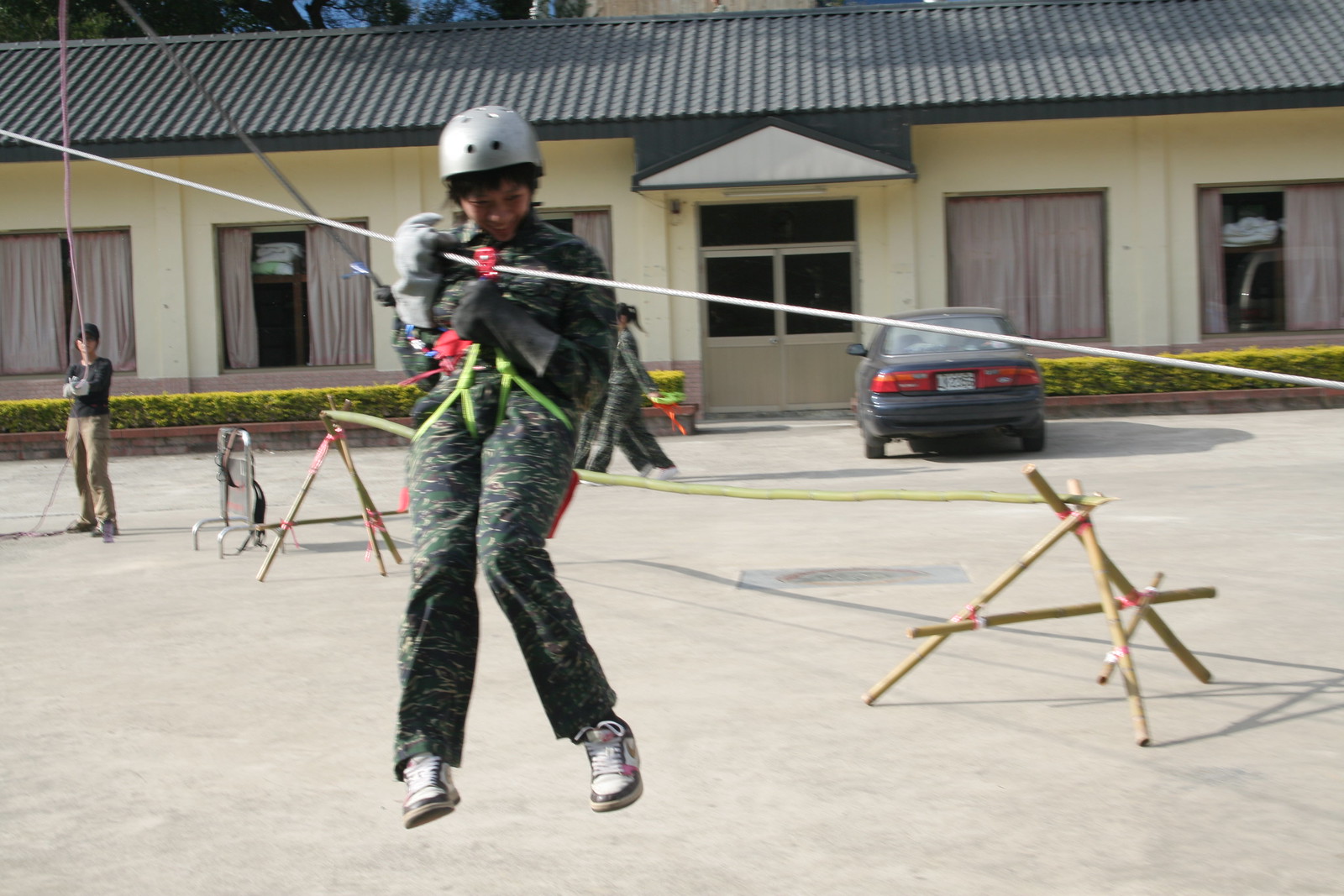A young girl, dressed in camouflage military fatigues, is suspended mid-air on a zipline, which is prominently positioned slightly above ground level. She’s equipped with a fluorescent green harness, a silver climbing helmet, and thick silver gloves, and she confidently holds onto the line while wearing tennis shoes. The background reveals a bustling scene set against a single-story building that could be a hotel or motel, identifiable by its silver roof with a turquoise outline, and large picture windows to the right. This building also features gray double doors at its center, with a green car parked directly in front of it. Nearby, some women clad in identical camouflage jumpsuits walk past the vehicle. Trees, some hedges, and a concrete lot with bamboo-style fencing cordon off the area. To the left, a person dressed in tan pants, a black shirt, and a hat, stands with arms crossed, while another figure holds a rope attached to the zipline, possibly assisting the ziplining girl as she navigates her descent. The overall scene suggests an organized outdoor event, with a hint of military training perhaps.